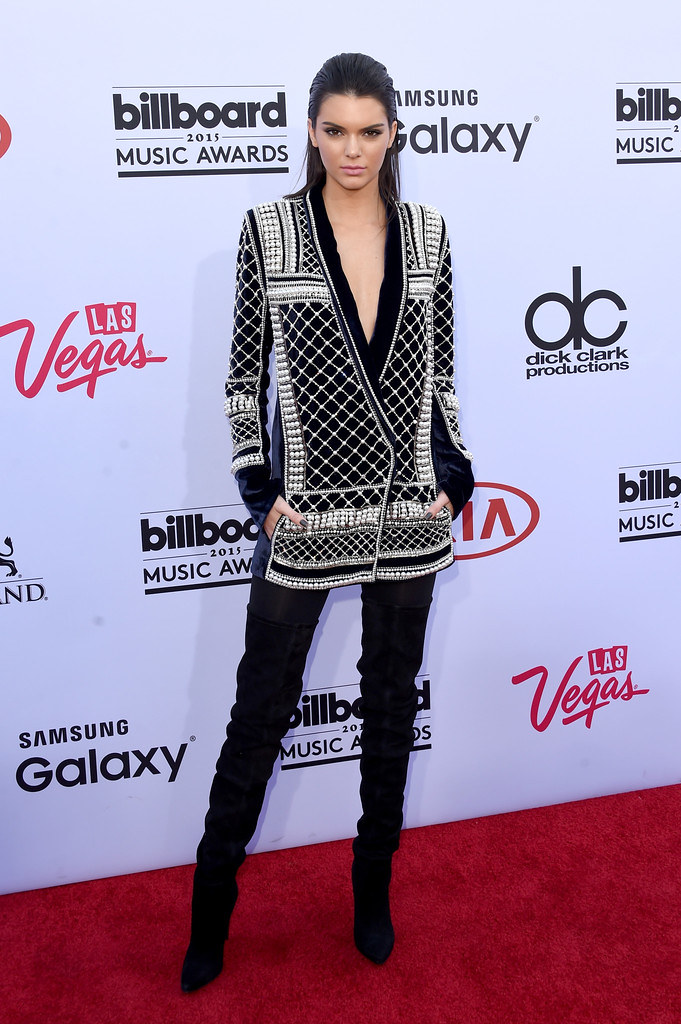The photograph captures a young woman with olive-toned skin and shoulder-length dark hair styled with part of it slicked back. She stands confidently on a red carpet, centered in the frame and facing the camera with a serious, neutral expression. Her outfit features a distinctive black and white, long-sleeved sweater or vest with a prominent V-cut neckline, revealing a black shirt underneath. The sweater showcases intricate grid and pattern designs along the arms and front. She pairs this with black trousers and black high-heeled boots. Her right leg is poised at an angle while the left remains straight.

Her hands are casually placed in her pockets, with thumbs resting outside. Behind her is a backdrop crowded with repeated logos and advertisements from prominent brands and events, including "Billboard Music Awards 2015," "Samsung Galaxy," "Dick Clark Productions," "Las Vegas," and "Kia," where some of the text appears in red and others in black. The white background accentuates these logos, and hints at the event's location in Las Vegas. Her understated makeup, featuring nude pink lipstick, complements her poised and composed demeanor.